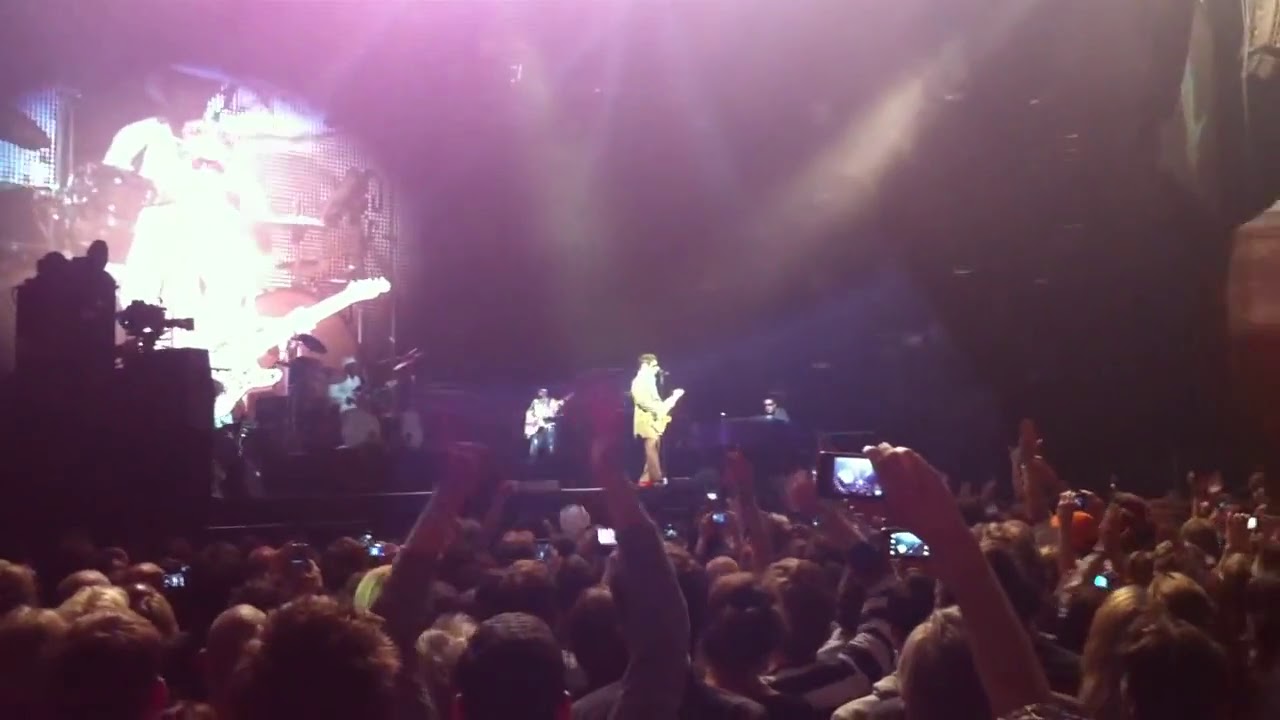This photograph captures a vibrant concert scene bathed in pinkish-purple lighting with a smoky atmosphere. Center stage, a man dressed in a yellow outfit, possibly a dress, sings passionately into a microphone while playing a yellow guitar. He sports sunglasses and has brown hair. Directly behind him stands another guitarist, while to their left, a keyboard player can be seen. The backdrop features a guitar emblem and a large drum set, adding to the musical ambiance. The stage, about six feet tall, is illuminated by strobe lights and bright yellow rays from the right, creating a dynamic visual effect. A large, enthusiastic crowd fills the foreground, many with their hands in the air and some recording the performance on their phones. To the left of the stage, a camera captures the concert, documenting this electrifying moment. The overall setting suggests a smaller, intimate venue, brimming with engaged fans.